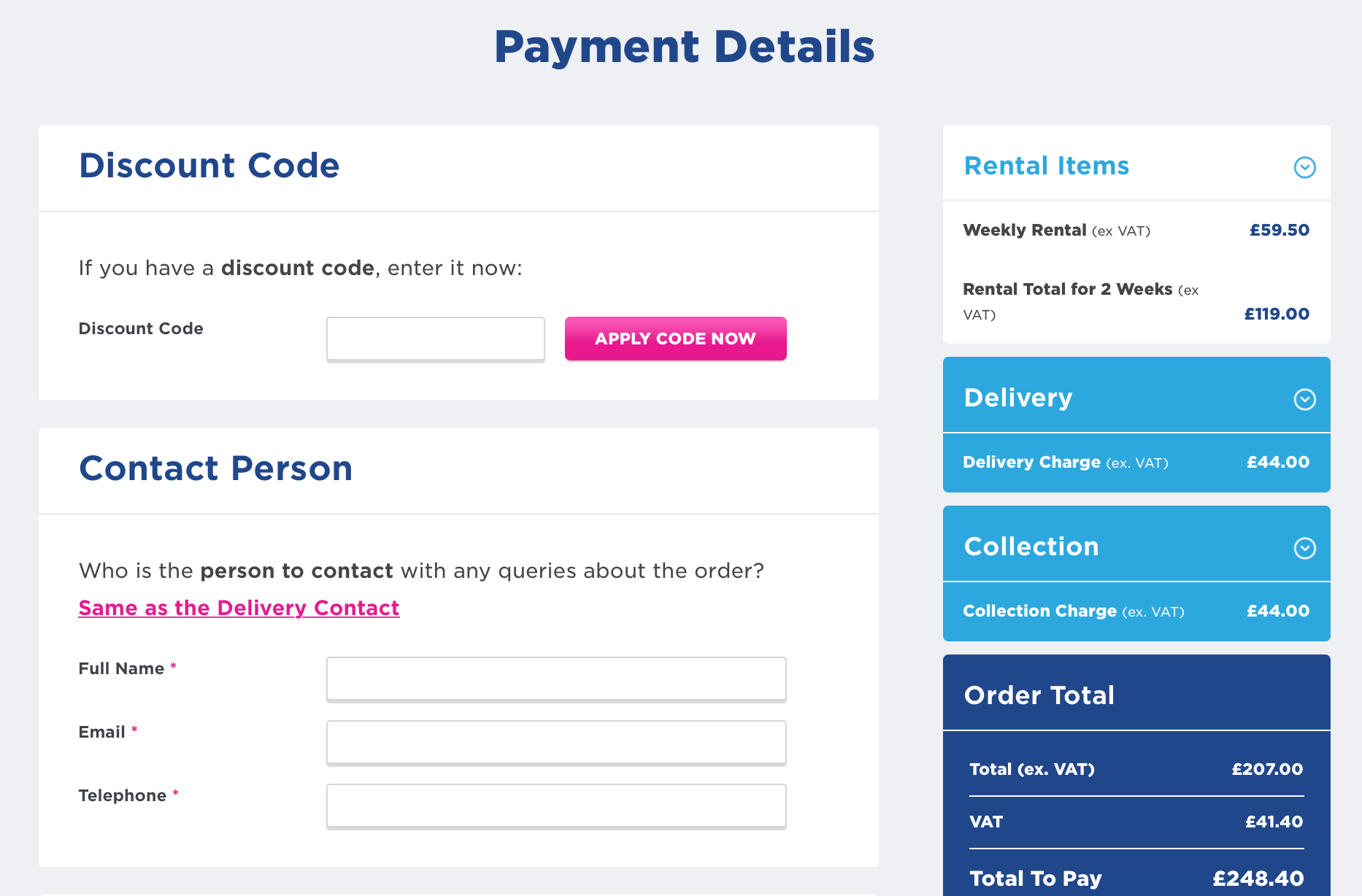The image displays an online payment details form for a business transaction. At the top, the title "Payment Details" is prominently highlighted in dark blue. Below this, there is a white box with a gray outline labeled "Discount Code," accompanied by a prompt: "If you have a discount code, enter it now." To the right, a pink box instructs users to "Apply Code Now."

Further down, the form requests the "Contact Person" information for any queries regarding the order. There is an option in pink, underlined, stating "Same as the delivery contact." Following this, there are fields labeled "Full Name," "Email," and "Telephone," each with a blank rectangle for input.

On the right-hand side of the form, a vertical column lists the rental item's financial details: 

- "Weekly renting, ex VAT: £59.50"
- "Rental total for two weeks, ex VAT: £119.00"
- "Delivery charge, ex VAT: £44.00"
- "Collection charge, ex VAT: £44.00"

The cumulative order amounts are also detailed:

- "Order total, ex VAT: £207.00"
- "VAT: £41.40"
- "Total to pay: £248.40"

Clarification notes are included at the bottom, explaining "ex" as excluding and "VAT" as Value Added Tax. The form does not provide any additional information beyond this.